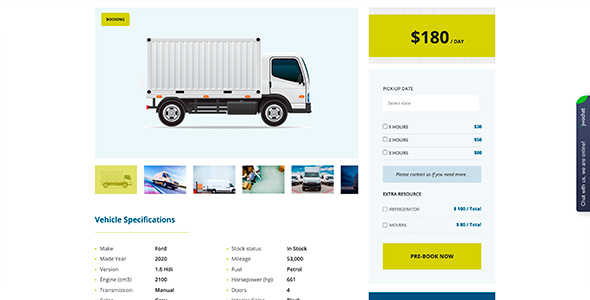A white Ford 2020 box truck is captured in motion, heading towards the right of the image, casting a shadow underneath it. The vehicle's front features dark-tinted windows and safety orange lights. Above the truck is a yellow rectangle displaying the word "Vehicle Specifications." The truck's detailed specifications are partially visible next to its image, listing it as a manual transmission model with a 2100 engine, 661 horsepower, and a mileage of approximately 53,000 miles. It is noted to be in stock and available for rental at $180 per day. Below the specifications, a form invites users to select their pickup date and rental duration, ranging from one to several hours. An "Extra Resource" option is available, and the bottom of the listing features a "Pre-book Now" button in a yellow rectangle.